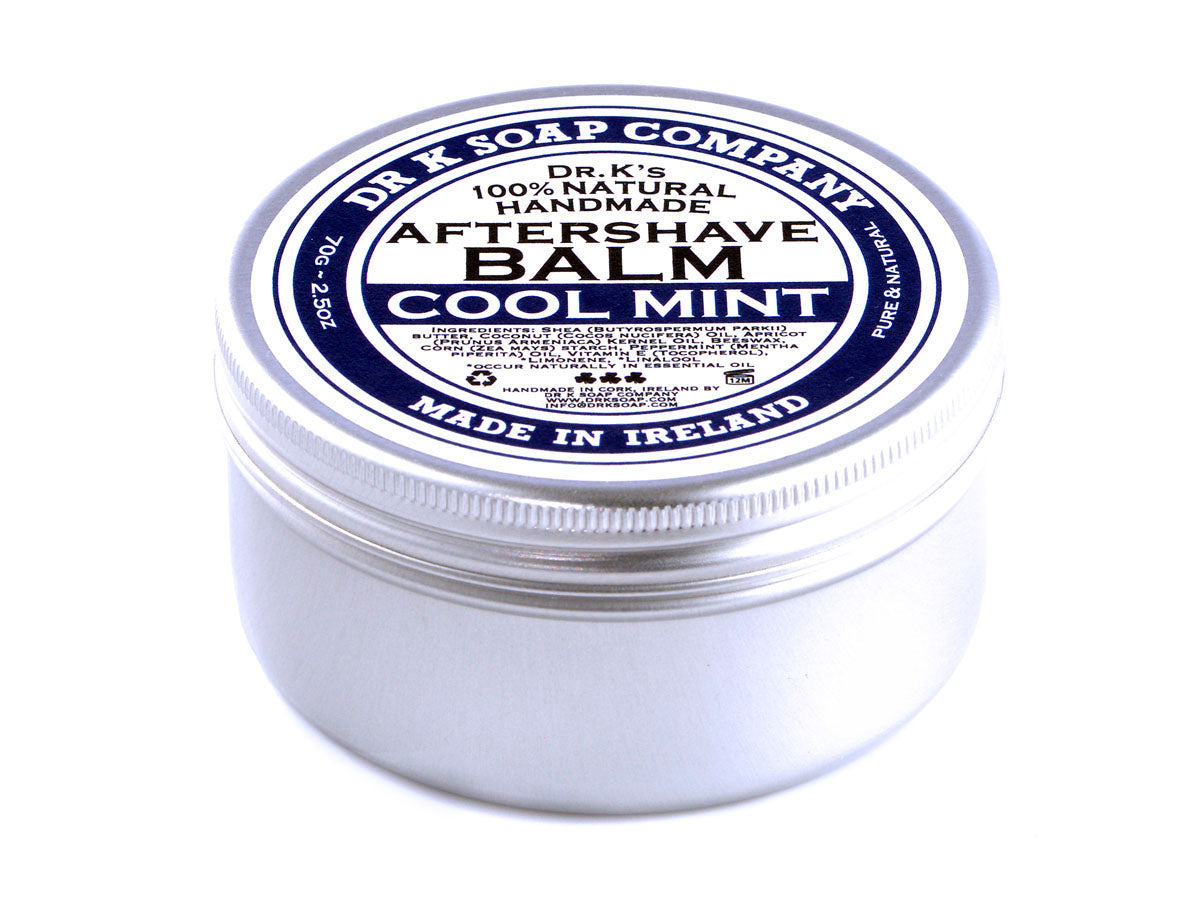The image depicts a small circular glass container with a silver, grooved spin-on cap. The body of the container is white and shallow. On the top, there's a prominent blue circle with white lettering that reads "Dr. K's Soap Company," and underneath, it says "Made in Ireland, Pure and Natural." Below this, in the middle section, there's a label with black text on a white background stating "Dr. K's 100% Natural Handmade Aftershave Balm Cold Mint." Surrounding these labels are additional details including a recycling symbol and an image of an oil can with its top popped open labeled "oil." Beneath the text, there are three small clover designs. There is also a small, illegible text below the main labels indicating potentially additional product information.